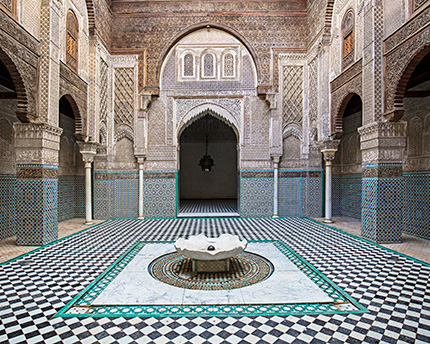This full-color square photograph captures an ornately designed indoor space with a rich, historical aura, suggestive of a religious building, possibly a mosque or cathedral. The foreground is dominated by a floor with black and white checkered tiles, infusing a classic touch. Elevated on a white marble pedestal at the center is a sculptural water fountain resembling a seashell, containing a distinctive black ball. Flanking the fountain are elaborate columns with striking blue bases, transitioning to arches of brown stone above. The arches form elegant walkways and hallways, contributing to a Middle Eastern architectural feel. At the far end, a pointed arch doorway crowned with lighting leads to another space, underscored by a series of smaller arched windows, adding depth and intricacy to the scene. The overall ambiance is one of timeless sanctity, combining elements of stone, tile, and decorative art.